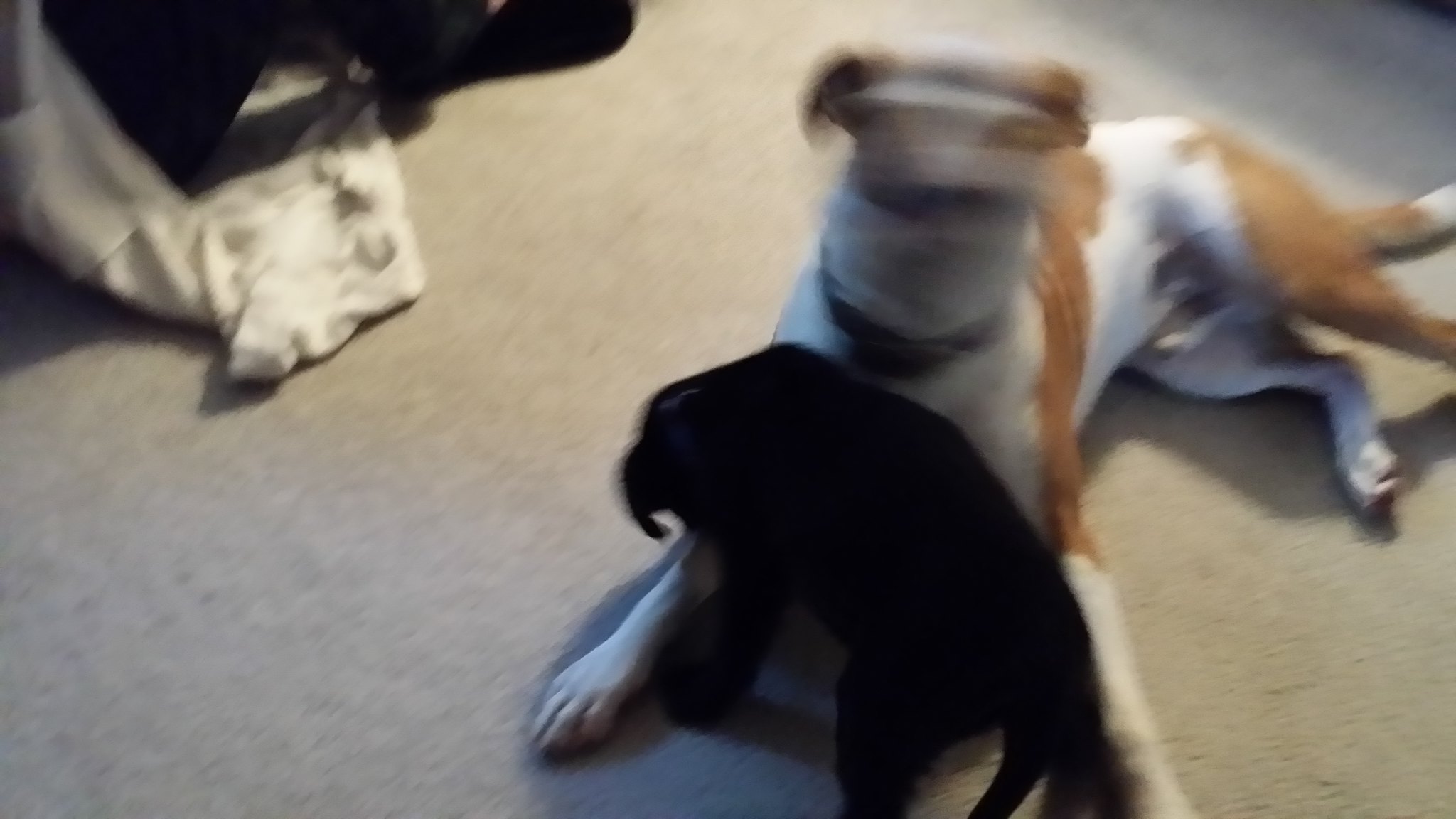The photograph is a very blurry, indoor, landscape-oriented image depicting two dogs on a pale gray, soft carpet in what appears to be a dark living room. The primary dog in focus appears to be a white and tan pit bull with short ears and some black patches. The pit bull is in the middle of shaking its head, resulting in a blurred face, and is wearing a black collar. Its pose shows its paws outward and a visible large brown patch on its back leg. Positioned in front of this dog, there is a smaller entirely black dog or puppy, characterized by a long tail and floppy ears. The background features some crumpled white clothes or sheets, and there are hints of furniture under a dim, yellowish overhead light, which illuminates the scene but does not brighten the room significantly.